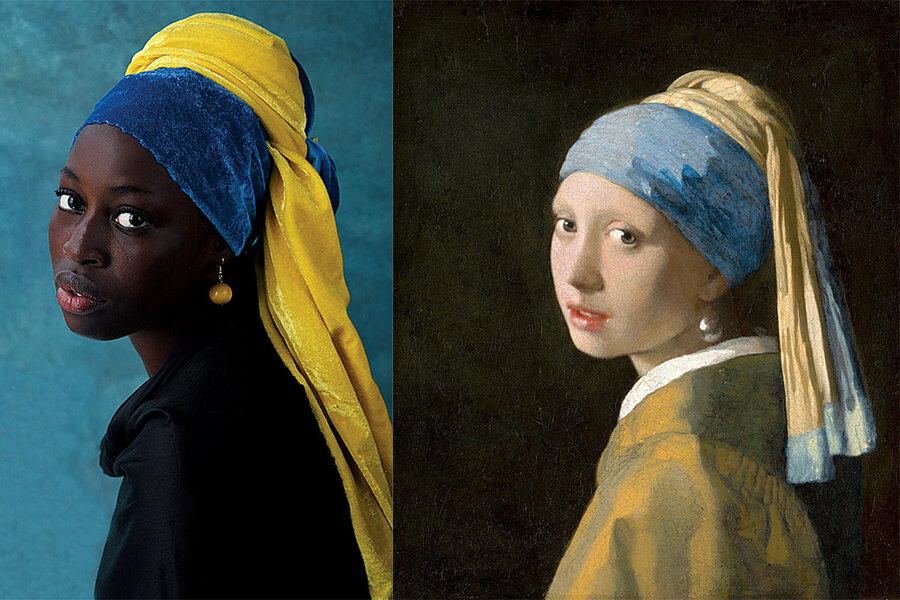The image showcases two side-by-side portraits of women set against distinctly colored backgrounds. On the left is a photographic portrait of an African American woman with a teal blue backdrop. She has minimal makeup and is adorned with yellow drop earrings and a prominent blue headband. The headband, which is followed by a yellow scarf draping behind her, accentuates her look along with a black shawl or shirt that gracefully covers her shoulders.

The right side features a painting of a Caucasian woman against a dark backdrop interwoven with dark gray and greenish hues. Her blonde hair is elegantly tied up with a blue headband, similar in style to the woman on the left, complemented by a cream-colored scarf tinged with blue that cascades behind her. She showcases a pair of silver drop earrings and has reddish lips that stand out against her light skin. Draped over her shoulders is a large robe with a white collar, colored in shades of orange and green, adding to the cohesive yet contrasting elements of the portraits.

Despite the different mediums—one being a photograph and the other a painting—and varying backgrounds, both women share a visually harmonious theme in their headbands and overall attire, blending traditional and modern aesthetics.